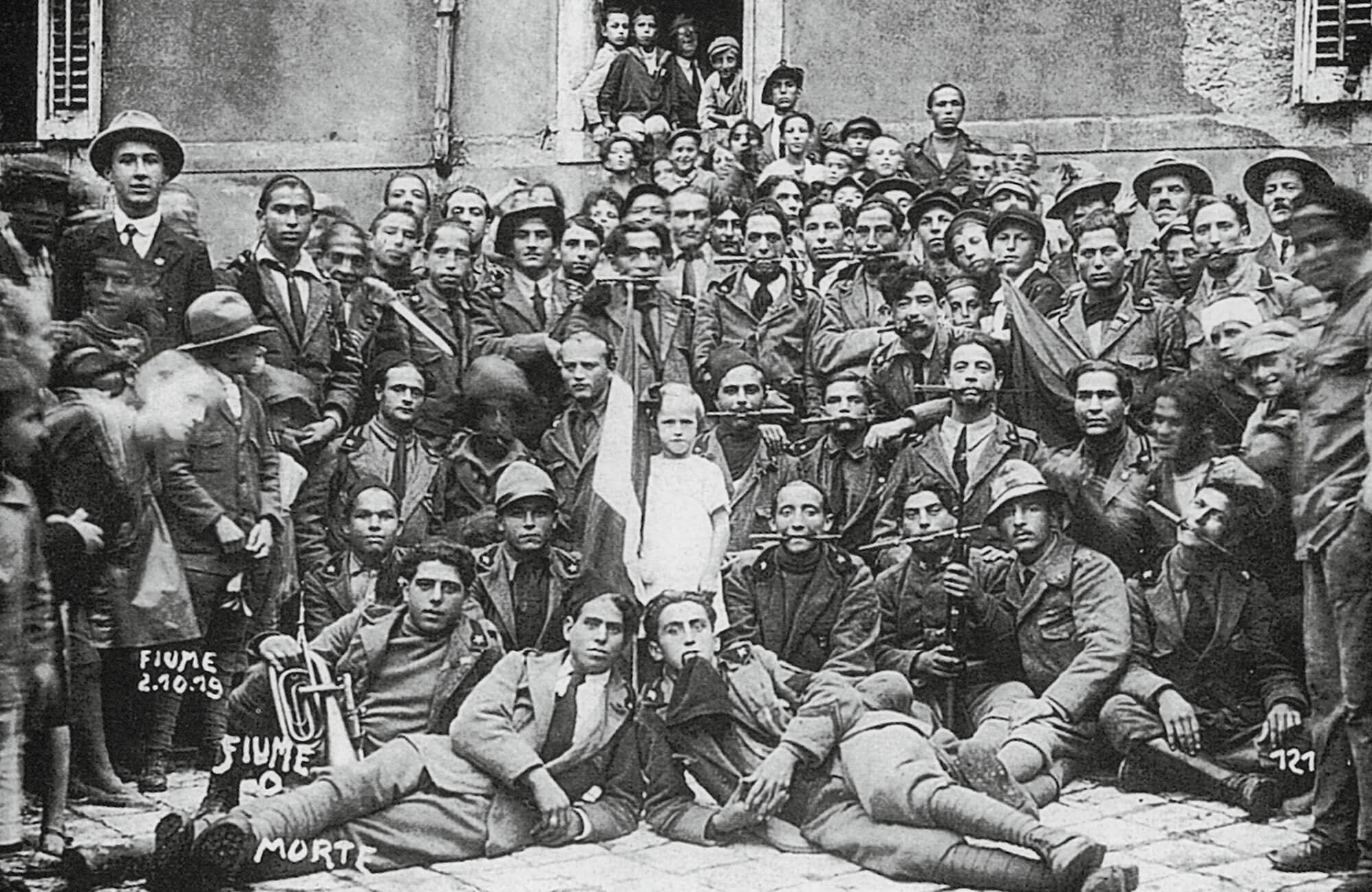This antique, black-and-white photograph, taken on 2.10.79 as noted by the handwritten "F-I-U-M-E" inscription in the lower left corner alongside a small heart, depicts a large, meticulously posed group of predominantly men in vintage suits. The men, some standing, kneeling, or even lying down, exhibit solemn expressions as they are densely packed in a circular formation against an old masonry wall with window blinds at both extreme ends. Centrally positioned is the solitary figure of a little girl in a white dress and bow, holding or draped with what might be a flag. Notably, several men in the middle have peculiar foot-long black tubes extending sideways from their mouths. The photograph emanates an air of solemnity, capturing not only the period attire but also the collective demeanor of the assembly.